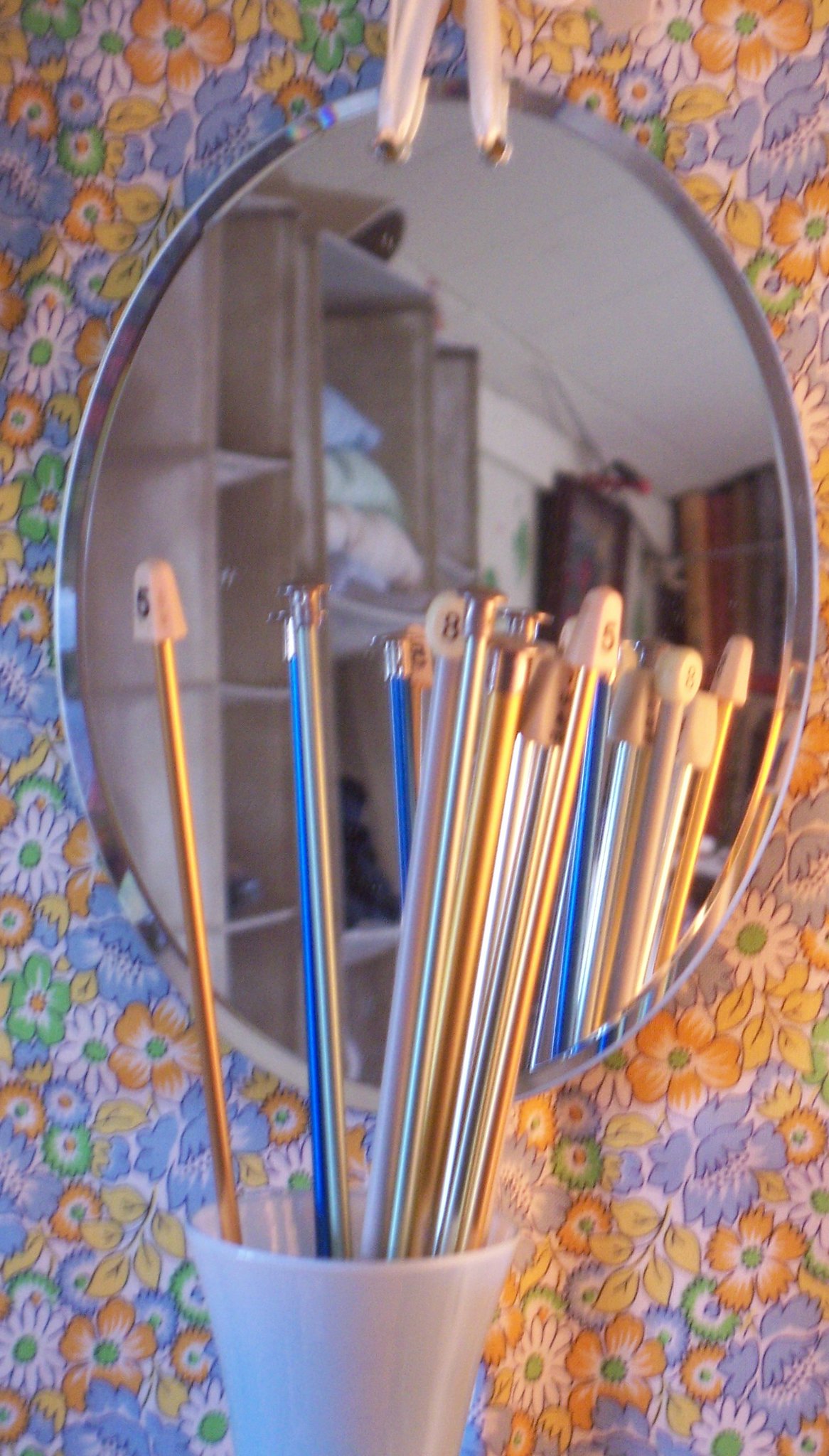The image features a vibrant floral wallpaper completely covering the background, densely packed with vividly colored flowers in shades of orange, blue, yellow, white, and green. At the center of this lively backdrop is a smaller, oval-shaped mirror held up by two grips or perhaps a white rope. Placed a little beneath the mirror is a white cup, containing several skinny metallic rods that resemble knitting needles or peculiar sticks. These rods, some gold, blue, and silver, are tipped with small wooden thimble-like shapes and marked with various numbers such as five and eight.

The mirror not only reflects these rods but also offers a glimpse into a room beyond, revealing large cabinets or shelving units that appear to be holding items like pillows and blankets, possibly in blue, green, and orange hues. The reflection is slightly distorted, making it difficult to precisely identify these items, but hints of yellow, brown, and red can also be seen in the background, along with a possible statue and a window.